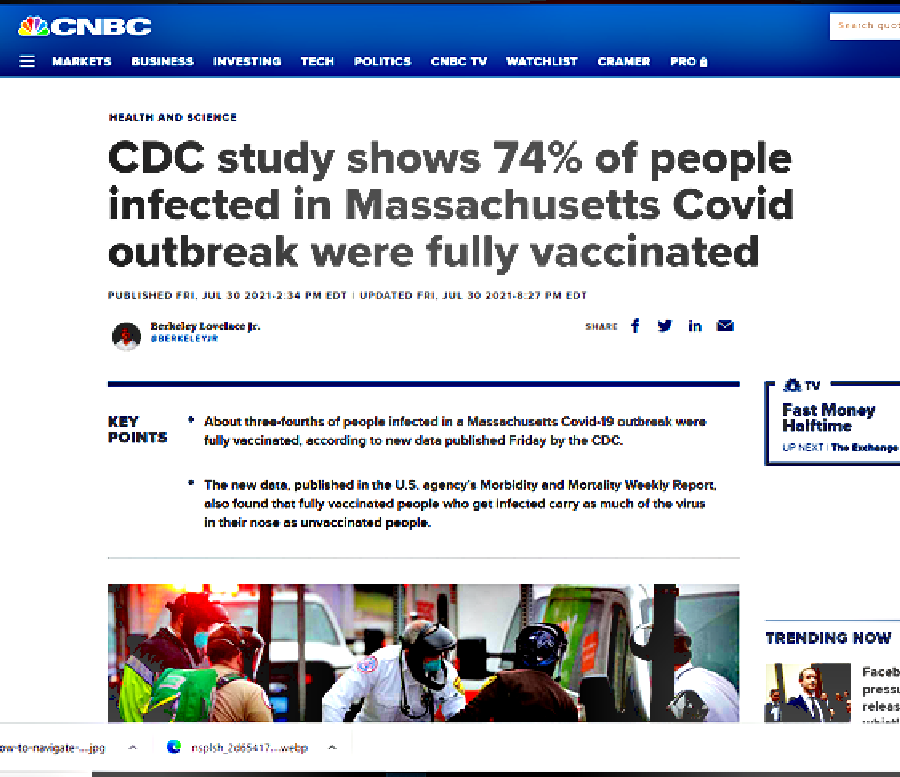Screenshot of a CNBC article webpage featuring detailed information and analysis of a CDC study on COVID-19 vaccinations and infections.

The top of the page is marked by a blue navigation bar, showcasing the CNBC logo adorned with the network's signature peacock symbol in white. The navigation menu includes categories such as Markets, Business, Investing, Tech, Politics, CNBC TV, Watchlist, Kramer, and Pro, alongside a white search box located on the upper right-hand side.

Below the blue navigation bar, the page's background is predominantly white. In small font, the subcategory "Health and Science" is displayed. The article's title is bold and large, reading: "CDC study shows 74% of people infected in Massachusetts COVID outbreak were fully vaccinated."

Beneath the title in smaller font, the publication details are noted: "Published Fri, JUL 30, 2021, 2:34 p.m. EDT. Updated Fri, July 30, 2021, 8:27 p.m. EDT." There's an icon suggesting an author profile, potentially of a black man, though the details are unclear. The name appears to be "Berkeley Landis Jr.," with a handle noted in blue.

Further down, social sharing icons are provided: an F for Facebook, a Twitter bird logo, IN for LinkedIn, and an envelope for email sharing. A dark horizontal line divides the sections.

Highlighted under "Key Points" are two bullet points summarizing the study's findings. The first bullet states that about three-fourths of individuals infected in the Massachusetts COVID-19 outbreak were fully vaccinated. The second bullet elaborates that the CDC's Morbidity and Mortality Weekly Report indicates that fully vaccinated persons who become infected carry as much viral load in their noses as those unvaccinated.

On the right side of "Key Points," a small box promotes the television schedule, noting "Fast Money Halftime" is up next, followed by "The Exchange."

Below the text, a striking image shows individuals wearing gas masks, with a couple of white vans visible in the background. To the right of this image, under a "Trending Now" section, a photo of Mark Zuckerberg accompanies the headline "Facebook press release."

The bottom of the image contains additional text that is too fuzzy to decipher, followed by another horizontal black line marking the page's end.